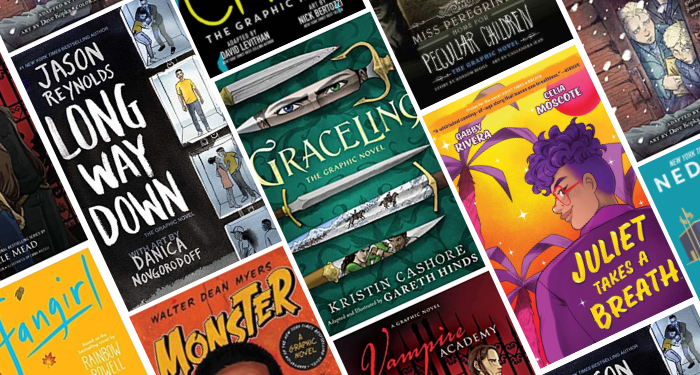The image depicts a collection of book covers arranged in angled, colorful squares with white lines framing them. Prominently visible are three book covers: "Long Way Down" by Jason Reynolds, featuring white text and four colored drawings of people on the right side; "Graceling" by Kristin Cashore, characterized by green hues and intricate sword imagery; and "Juliet Takes a Breath" with vibrant yellows and reds, showcasing a cartoon figure with curly purple hair and red glasses. Parts of other book covers, such as "Vampire Academy" and indications of titles including "fangirl" and "monster," are scattered around the periphery, partially cut off by the image's borders, adding a dynamic, layered visual effect to the scene.